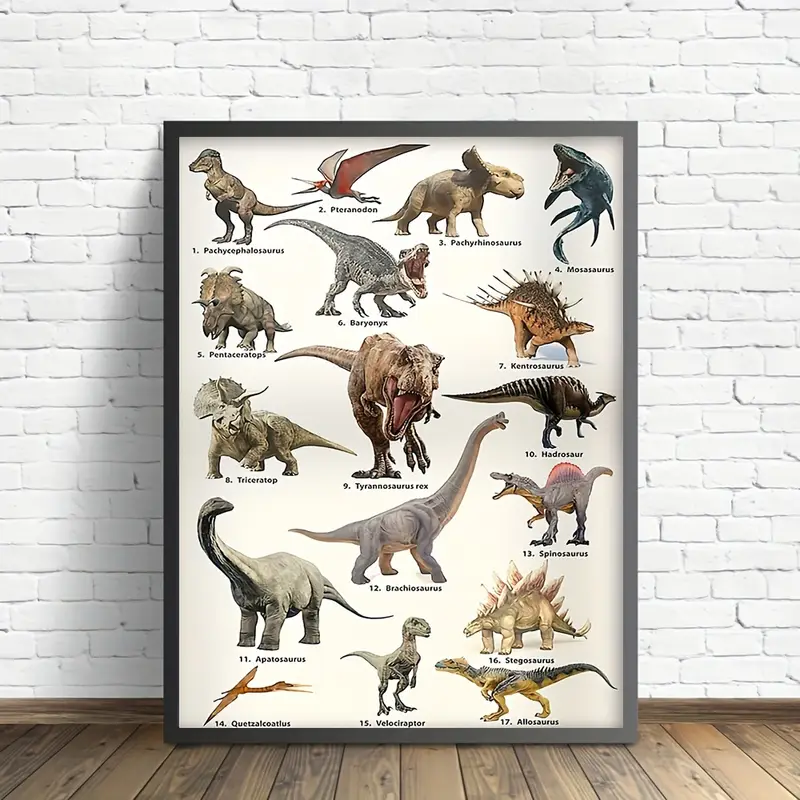The image captures a detailed color photograph of a framed poster, presented in a vertical portrait orientation. The poster, adorned with a dark gray wood frame, leans against a whitewashed brick wall, with a light brown wooden plank floor beneath it. The subject of the poster is a meticulously illustrated collection of prehistoric dinosaurs, each depicted in realistic, representational detail. The illustrations are numbered and labeled, showcasing a variety of dinosaurs found on land, in water, and in the air. Prominently, in the center, is a T-Rex, easily identifiable with its mouth wide open. Surrounding the T-Rex are approximately 15 other dinosaurs, arranged in what appears to be a random fashion of rows and columns. Detailed depictions include a tall dinosaur with a long, pointy tail and short front legs on the top left and a dinosaur with two long red rings and an open beak to its right. The overall scene is set against the backdrop of the wooden slat floor and white brick wall, framed by the gray and black trim, contributing to the photograph's realistic and richly descriptive composition.